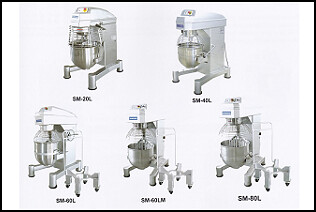The small image showcases five stand mixers, likely depicted in light gray photographs with a silver-gray tone, arranged in two rows—two on the top and three on the bottom. Each mixer has a hooded body and a large mixing bowl in the front, along with short cylindrical legs that have black rubber pieces on their feet. These legs are connected by horizontal cross members for stability. Distinguishing features between the mixers are difficult to ascertain due to the photo's clarity, but they appear similar in design. Underneath each mixer, there are tiny, blurry model numbers in black text, suggesting that this image might be from a catalog or an online store. Rendered in grayscale with a simple, white background and a thin black border, the image includes vertical white stripes on the left and right edges.